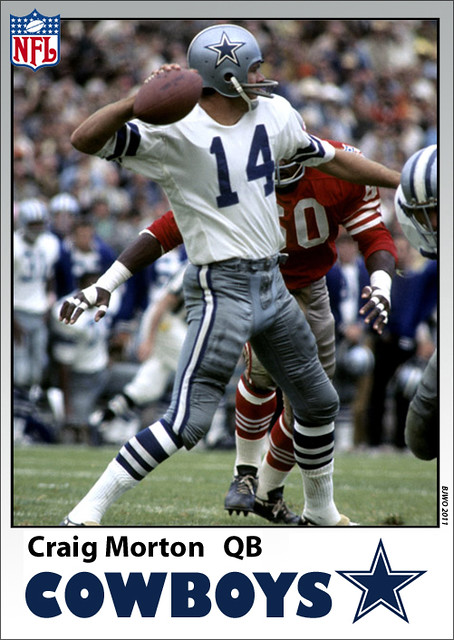This image showcases a vintage football card featuring quarterback Craig Morton of the Dallas Cowboys. Morton is depicted in action, seemingly poised to throw the football he holds in his right hand. He is wearing a white jersey with blue number 14 and gray pants accented with a blue and white stripe along the sides. His helmet is gray with a prominent blue star. The card's design includes a blue border, with the NFL logo in the upper left corner. Below his image, 'Craig Morton QB Cowboys' is labeled in blue text next to a blue star. Another detail includes a black text inscription on the right side that reads 'BJ WO 2011'. The overall appearance of the card suggests it is quite old, likely dating back to Morton's playing days before the era of Tony Romo. The background hints at imminent action as Morton appears ready to evade a potential tackle, possibly from a player on the 49ers.